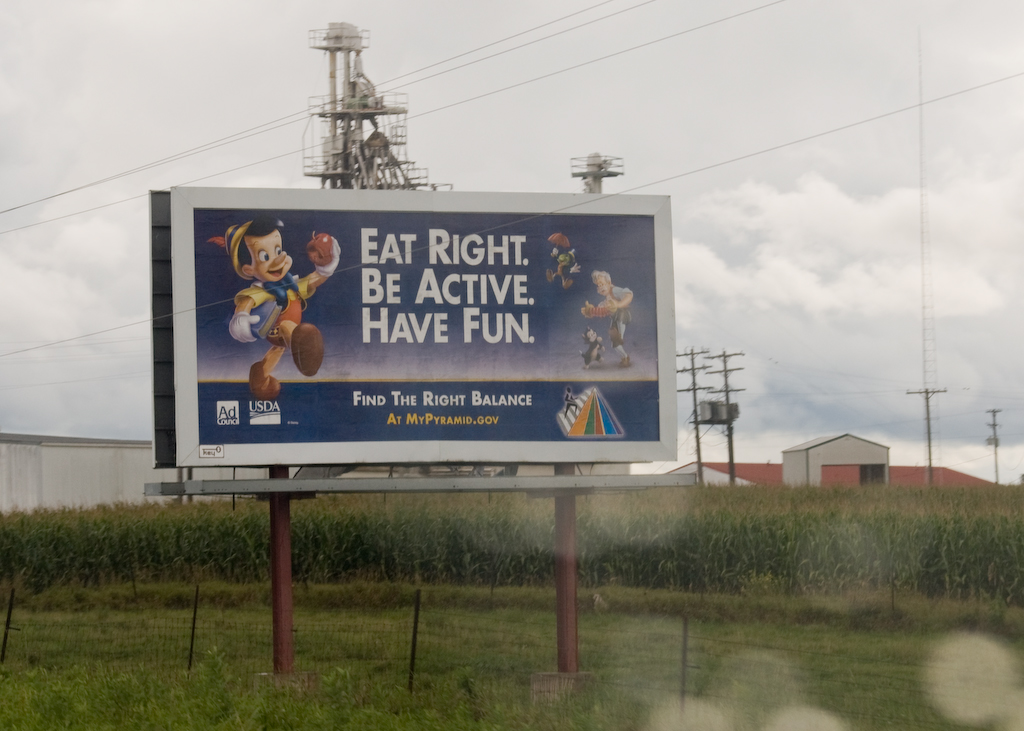Here is a refined and detailed caption for the image:

"Nestled in a vast tarpaulin field, a prominent billboard stands tall against a backdrop of a lush cornfield. The billboard, advertising a movie featuring characters Pinocchio and Geppetto, bears the uplifting message: 'Be Active, Have Fun.' In front of the billboard, a black wire fence delineates the immediate grassy section of the field from the advertisement. The top of the cornfield is visible in the background, slightly elevated, creating a layered landscape. Off to the left, partially obscured behind the cornfield, a quaint house adds a touch of rural charm to the scene."